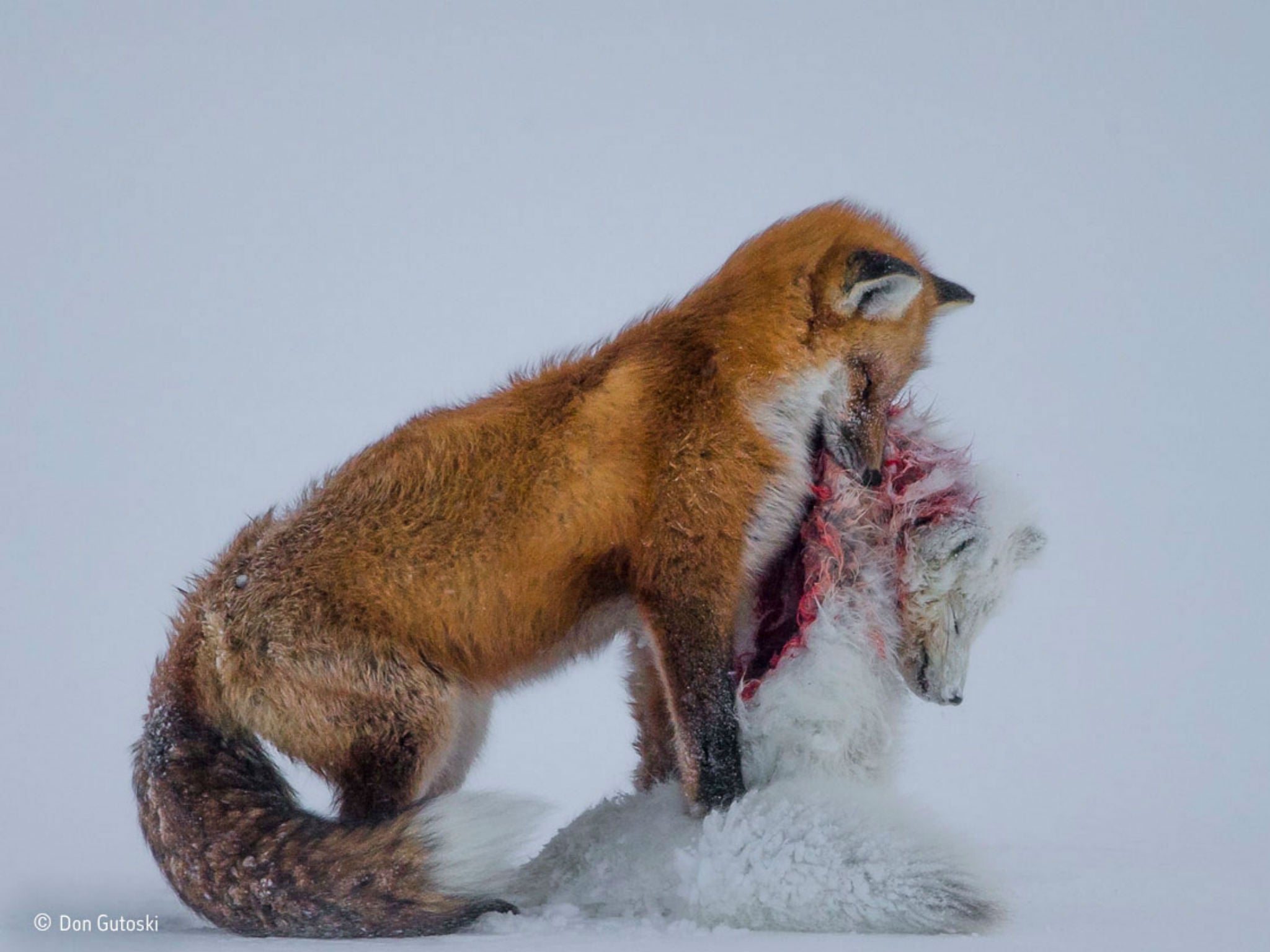This color photograph, taken by Don Gutosky, features an evocative and intense wildlife scene set against a pale blue background that seems almost empty, highlighting the starkness of the moment. Dominating the center of the image is a brown fox, characterized by its large bushy tail, with black-tipped ears, tail, and legs, which is curled up in front of it showing some snow on the tail. The fox's eyes are closed as it holds the lifeless body of a smaller, white fox in its mouth, its head hanging downward to the right. Blood is smeared on the body of the white fox, indicating a recent kill. The scene captures the raw reality of nature and underscores the predatory instincts of the fox. The photograph's quiet background draws full attention to this poignant moment, with the copyright text "Don Gutosky" discreetly positioned in the lower left corner.